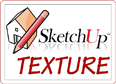The image depicts a photorealistic, textured surface resembling a slab of marbled paper. The colors transition from almost white to light beige, tan, and medium brown, with numerous intricate lines and natural shapes giving the surface a mottled appearance. At the center of this marbled background is a watermark consisting of a simple but detailed drawing of a small house with a peaked roof, complete with a door and window. Overlaying the house is a large penciling sketch. Surrounding the central image in a circular fashion is the text "SketchUpTextureClub.com," with the watermark letters appearing intermittently across the marbled surface.